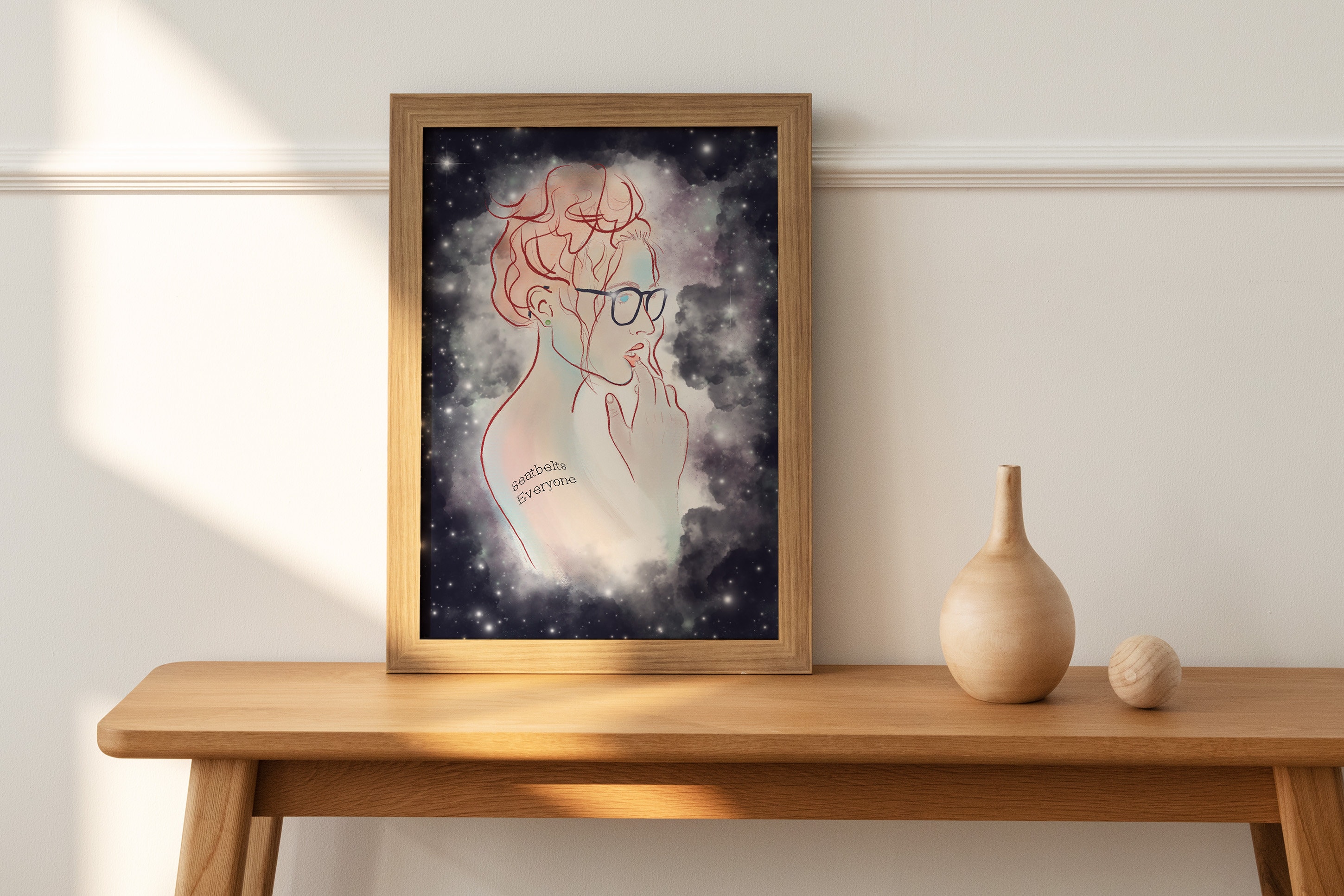The image presents an interior room scene featuring a light brown wooden bench against a light gray or possibly off-white wall with horizontal molding. Sunlight highlights the left side of the wall. The bench displays three main objects: a painting, a light brown vase with a very thin neck resembling a pottery urn, and a wooden ball.

The painting, framed in wood, depicts a female cartoon character with black glasses and pinkish-red or salmon-colored hair styled in a bun. The woman, positioned against a starry black background suggesting a nebula, holds a finger to her lips and has the phrase "seatbelts everyone" tattooed on her arm. Her gaze is directed off to the right. The artwork combines elements of outer space, represented by white spots that mimic stars, with the vibrant, graphic depiction of the woman, creating an interesting and artistic centerpiece for the scene.